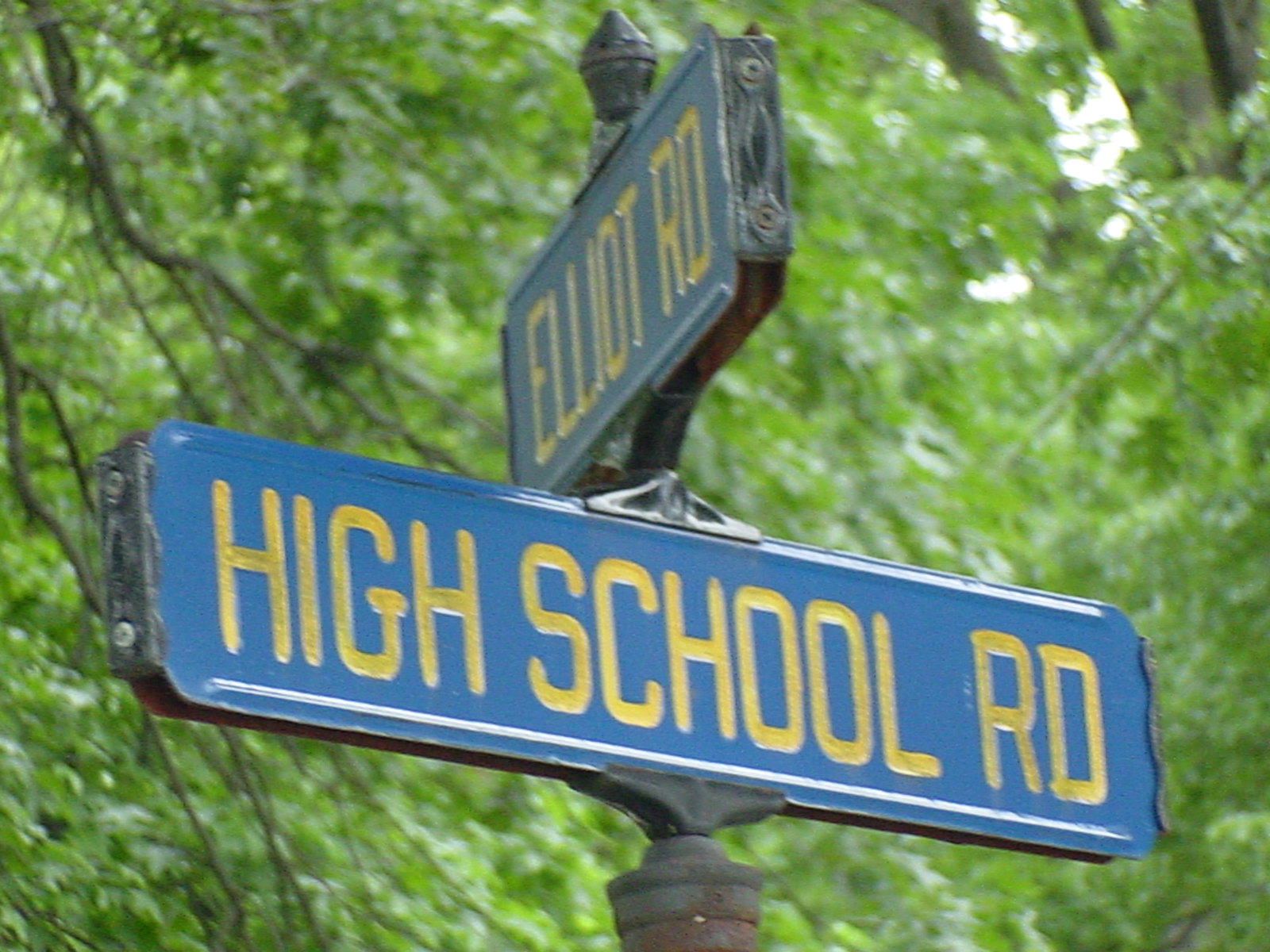In this zoomed-in photograph, the viewer's focus is drawn to a set of street signs mounted on a rusted pole. The background consists entirely of dense, wooded trees, emphasizing the natural, serene surroundings. The pole itself is visible from the top, which culminates in a pointed, bronze or silver tip. Two prominently placed blue signs with yellow letters indicate street names: the one facing the viewer reads "High School RD," while the sign positioned perpendicularly displays "Elliot RD" or "Elliot Road."